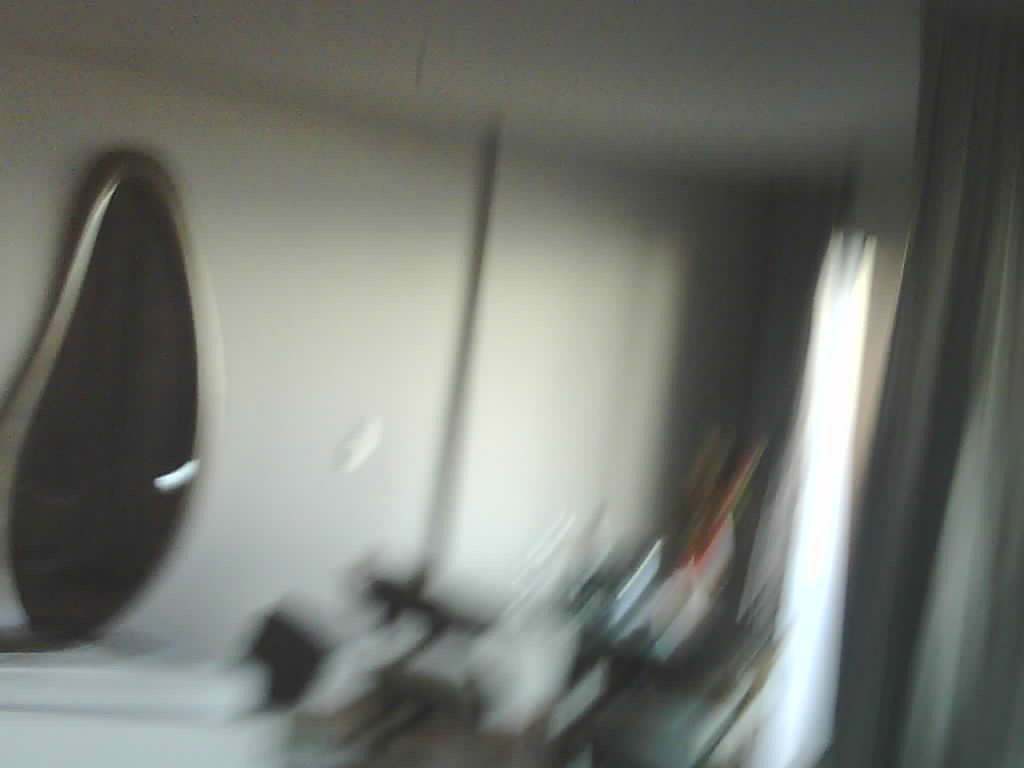In this photograph, likely taken in haste or accidentally while in motion, the image is extremely blurred. To the left side, a distinctive teardrop-shaped mirror with a gold frame is leaning against a white-painted wall, adding a touch of elegance. This setting seems to suggest the interior of a hotel room. On the right, window blinds and dark gray-brown curtains obscure potential outdoor views, allowing minimal light into the room. Dominating the center of the image is a large, indistinct shape, potentially a suitcase or a piece of exercise equipment, featuring a horizontal black metal bar with hints of red. The overall lack of clarity leaves much to the imagination, but the few visible elements hint at a cozy yet tastefully decorated space.